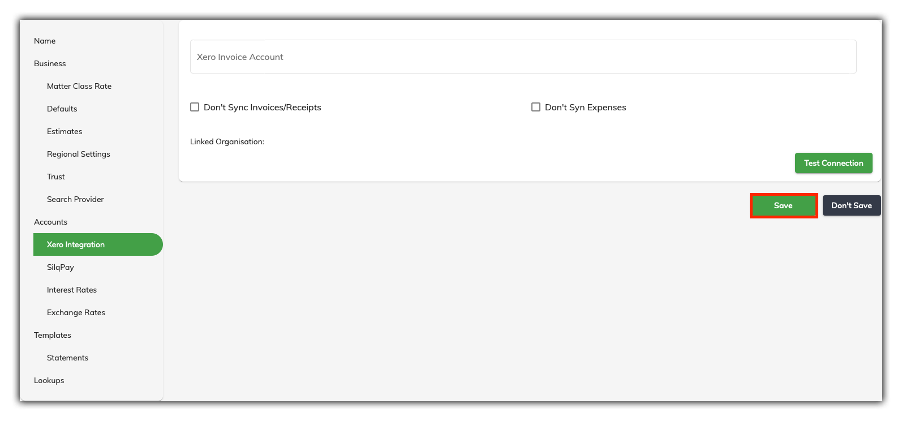This image captures a screenshot of a well-organized web page, which presents various sections and categories in a structured manner. The background of the page is a light gray rectangle, creating a neutral backdrop for the text content. 

At the top of the page, the word "Name" is prominently displayed in bold black print. 

Progressing downward, the section labeled "Business" serves as a header for a list of six detailed categories, each slightly indented:
1. Matter
2. Class
3. Rate
4. Defaults
5. Estimates
6. Regional Settings

Continuing further down on the left side, reverting to non-indented headers, the "Accounts" section appears. Within this, four specific areas are indented:
1. Xero Integration (highlighted with a green, curved rectangle)
2. Silo Pay
3. Interest Rates
4. Exchange Rates

Below this, at the non-indented level again, "Templates" is listed, followed by indented sub-category "Statements", and then returning to non-indented with "Lookups".

In the middle of the screen, a white rectangle area is shown containing interactive buttons: a green "Text Connection" button, a green "Save" button, and a black "Don't Save" button. These elements collectively illustrate the page's functionality and user options.